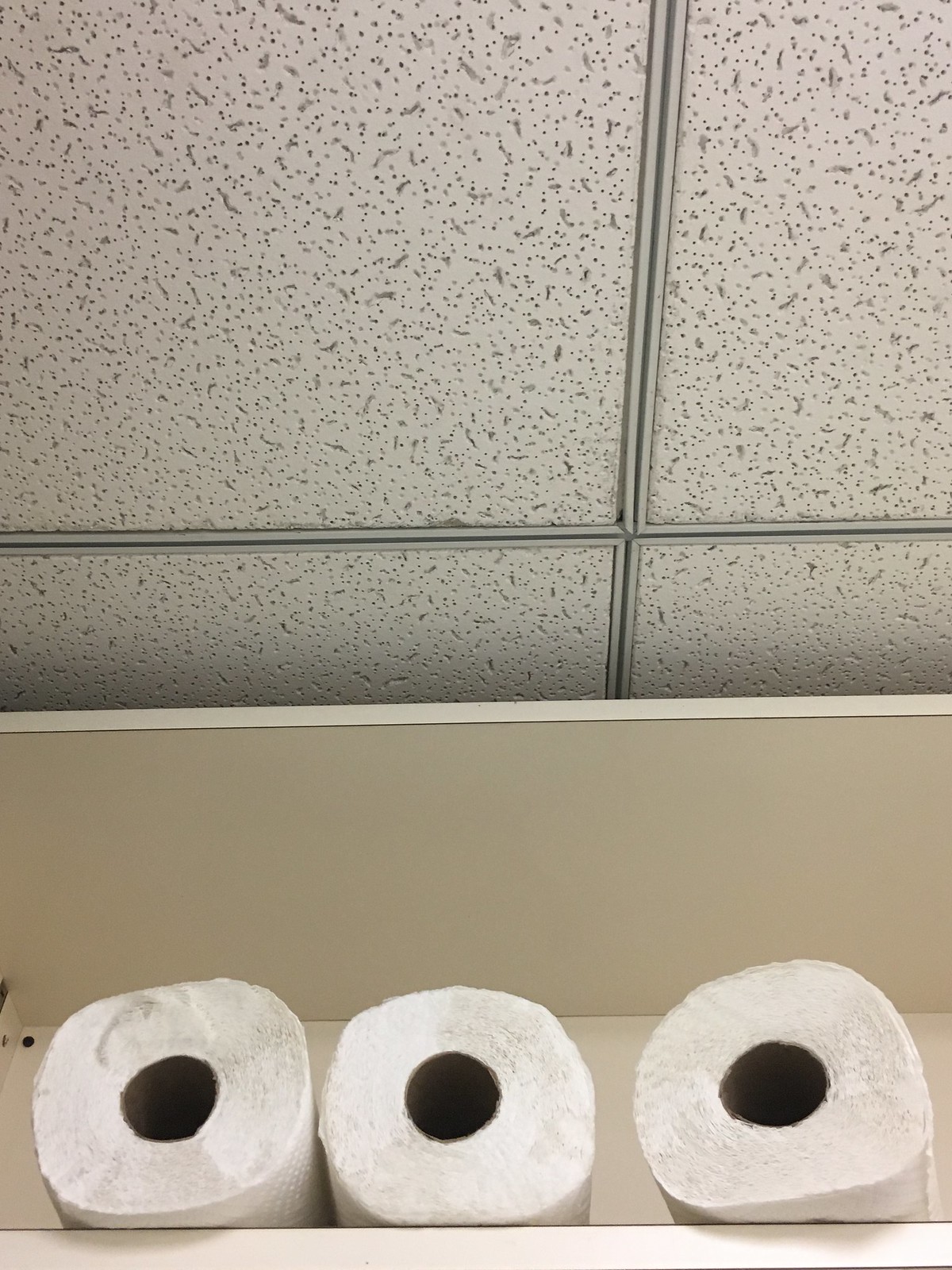The photograph captures a portion of a room, primarily focusing on a tall, white shelf positioned almost flush with the ceiling. The shelf, located in the lower half of the image, holds three rolls that appear to be paper towels, their ends facing outward. These rolls are notably deformed, suggesting they might be damaged, with wavy and smashed appearances that deviate from their usual round shape. Above the shelf, the ceiling dominates the upper half of the photograph, composed of large white tiles with silver metal grid lines dividing them. The tiles feature a textured surface with swirls and small holes, adding a subtle depth and pattern. The perspective of the photo is from a low angle, looking up at the shelf and the ceiling, which emphasizes the height of both elements and reveals the simple, yet detailed materials and textures present in the room.